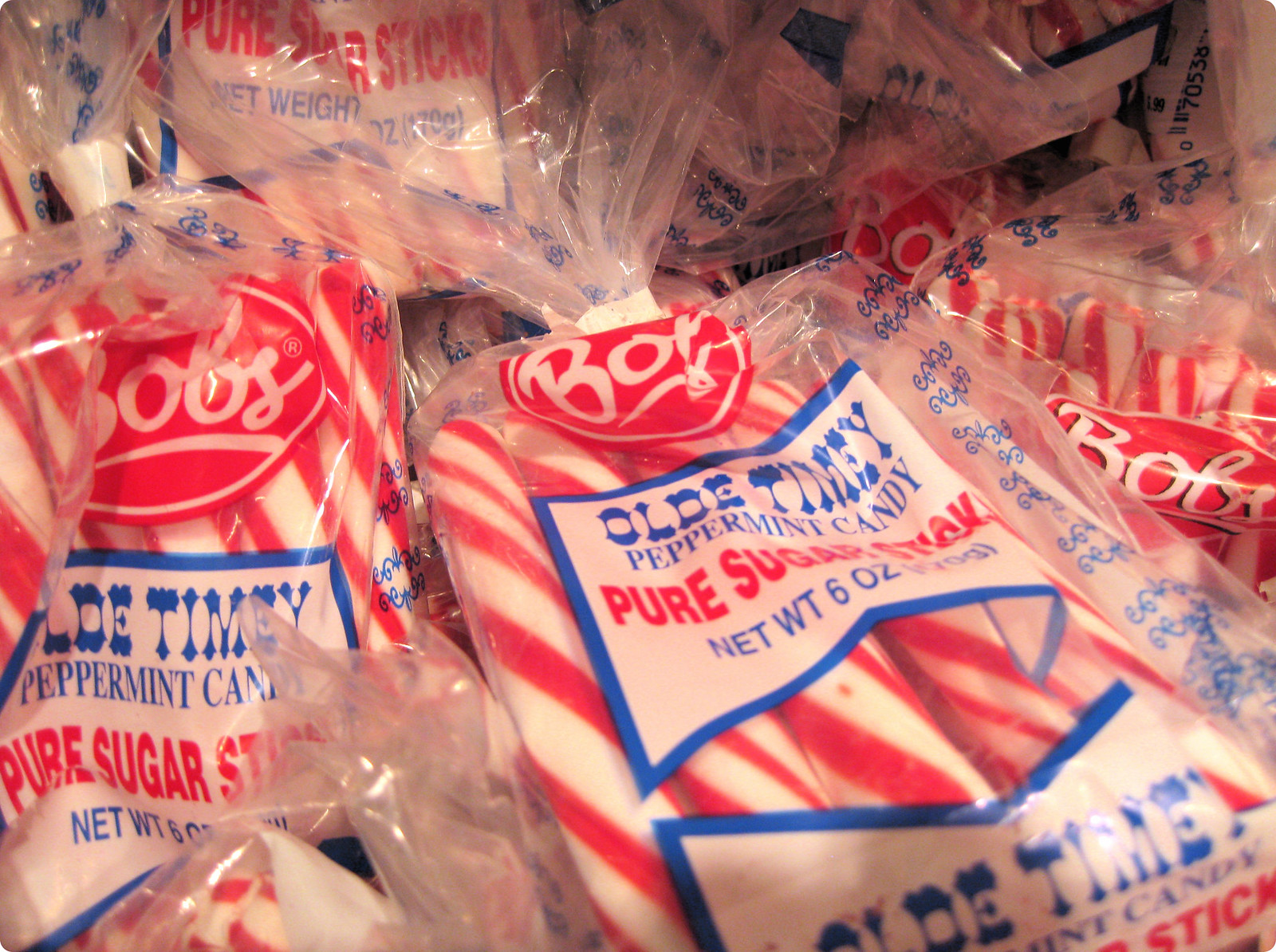The image showcases an abundant pile of clear plastic packages filled with red and white striped peppermint sticks stacked atop each other, completely filling the frame. Each package prominently features a red logo at the top reading "Bob's." In the middle of the package is a blue-bordered rectangle containing the text: "Old-Timey Peppermint Candy, Pure Sugar Stick, Net Weight 6 ounces, 170 grams." These peppermint sticks resemble the straight part of candy canes. The consistent design is noted across all the packages, emphasizing the brand and product details uniformly throughout the pile.